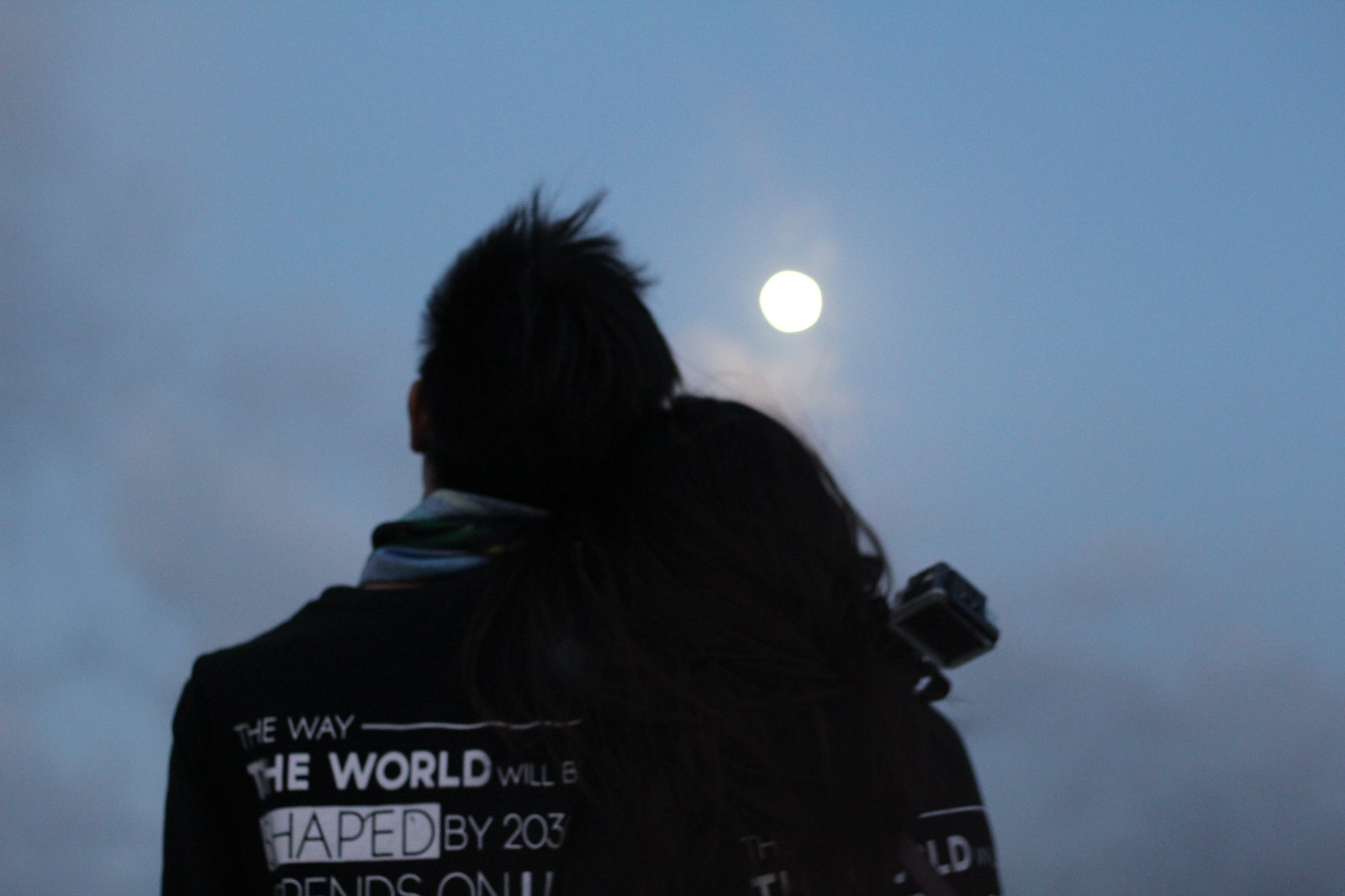This is a photograph of a couple standing outdoors, gazing up at a full moon that dominates the center of the image against a dusky, grayish-blue sky. The couple appears to be young adults, possibly in their teens to 30s, identified by their full, black hair—his short and hers long, extending to her shoulder blades. They are wearing matching black jackets with white text on the back. The text on the male's jacket reads in varying fonts and sizes: "The way the world will be shaped by 203- depends on." This text is partially obscured, but similar text is also on the female's jacket, though her hair covers much of it. Positioned to the right of the girl, there appears to be a GoPro or similar equipment, suggesting someone is holding it. Dense fog or clouds add a smoky appearance beneath the moon, enhancing the image's atmospheric quality. The couple appears close, perhaps hugging, and the entire scene evokes a feeling of quiet intimacy set against a twilight sky.